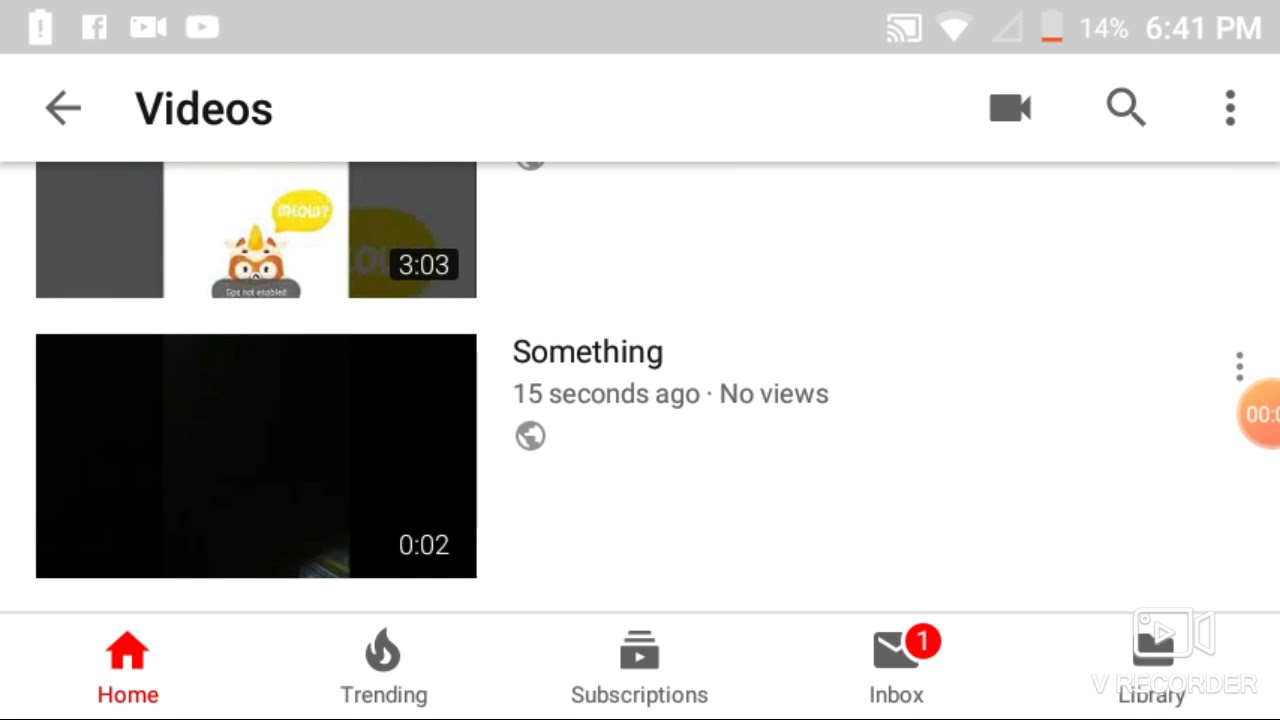A heavily cropped screenshot captures a smartphone screen displaying the YouTube app's main interface. Only a small section of the video previews at the bottom is visible, showing one video titled "Something," which is two seconds long and predominantly dark except for a slight illumination in the bottom right corner. This video was uploaded just 15 seconds ago and has no views.

Above this, another video with a thumbnail featuring a cartoon animal is partially visible, though its description is cut off. The YouTube app's bottom navigation bar is also visible, with icons for Home, Trending, Subscriptions, Inbox, and Library. Notably, the Inbox icon indicates one unread notification.

In the bottom right corner, a watermark reads "V Recorder," suggesting the image might be a screenshot or a recorded clip. The device's battery is critically low at 14%, with the time displayed as 6:41 PM. The background of the app and the interface is primarily white.